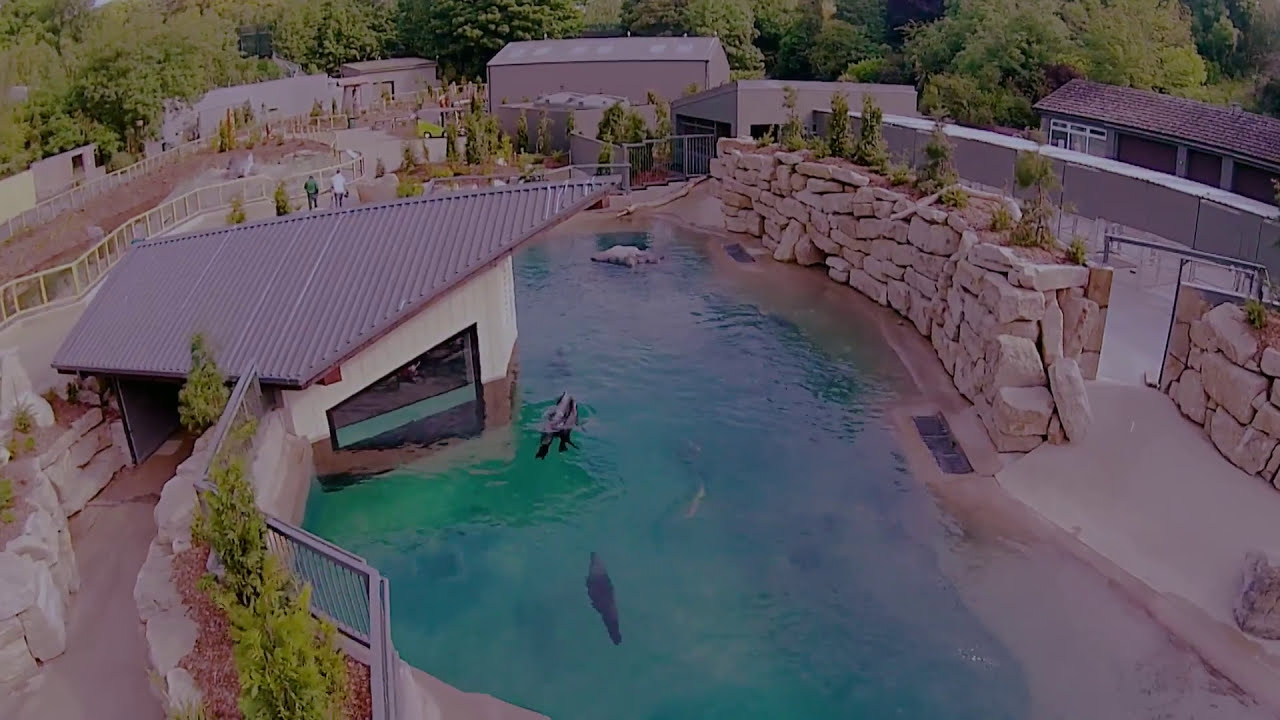The aerial view captures an outdoor aquarium holding tank, featuring a small blue pool occupied by several seal-like creatures. Two of these marine animals are visible underwater, while one is breaching near a partially submerged observation hut. The hut, distinct with its white upper walls and tan brick base, features a slanted metal brown roof and large windows, including one underwater window for close observation. A walkway behind the hut provides access and viewing opportunities for visitors. The pool is surrounded by tall stone walls, with a slotted gray fence on the left side, presumably where visitors walk, and a border of large white rocks on the right. Two people, one in a green shirt and one in a white shirt, are seen walking towards the back buildings adjacent to a forested area. The pool's water appears clean and serene, enhancing the naturalistic setting of this well-maintained aquatic exhibit.